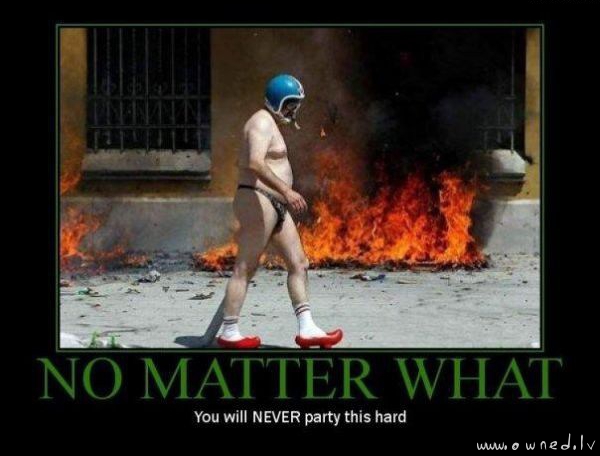In this humorous and chaotic meme, an older, out-of-shape man wearing a blue football helmet and an ill-fitting black g-string stands in profile. His absurd outfit is completed with white crew socks featuring red stripes and vibrant red high-heeled shoes. The surreal scene is set against the dramatic backdrop of a burning building, its walls engulfed in flames that send plumes of black smoke skyward. The building has two barred windows, one of which is partially obscured by the thick smoke. Debris is scattered around the fire's base, adding to the scene's havoc. Despite the surrounding destruction, the man appears nonchalant, embodying the image's caption: "No matter what, you will never party this hard." A website, www.WNDlive, is noted in the bottom right corner, further emphasizing the meme's satirical nature.